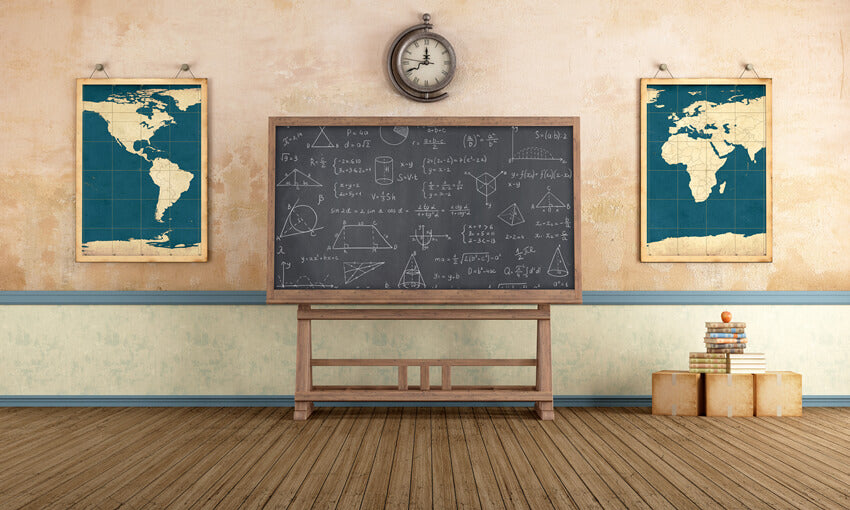In a modern yet old-fashioned classroom, the room's focal point is a large, dark gray chalkboard filled with an array of diagrams and equations, including geometric figures like pyramids, triangles, circles, and parallelograms, all intricately drawn in white chalk. The chalkboard is encased in a wooden frame with wooden legs. Flanking the chalkboard are two large, framed maps: on the left, a map of the Western Hemisphere featuring North and South America and Greenland in light yellow against a blue ocean, and on the right, a map of Europe, parts of Asia, and Africa in similar colors. Above the chalkboard, a quaint, old-fashioned clock is prominently displayed. The classroom walls are light orange and white, accented with blue and white trim, giving it a slightly aged, worn look. The wooden floor adds a modern touch with new wooden planks. To the right of the chalkboard, three stacked boxes hold multiple books, crowned with a single apple, adding a touch of traditional classroom charm.